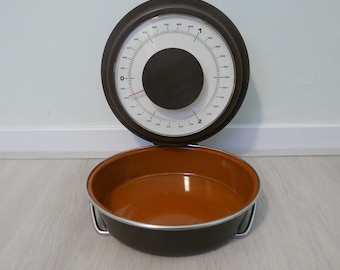The image showcases a detailed view of a round, metal kitchen scale positioned in front of a light blue wall and resting on a light beige floor. The scale features a substantial black circular rim and a central black circle, which is surrounded by a white ring displaying black measurement markings. Below the scale sits a shiny, metallic pan, which is black on the outside and has a brown interior. The pan also has silver handles on either side. The overall scene hints at a clean, modern kitchen setup, accentuated by the reflective sheen of the metal, suggesting its potential use for precise cooking or baking measurements.